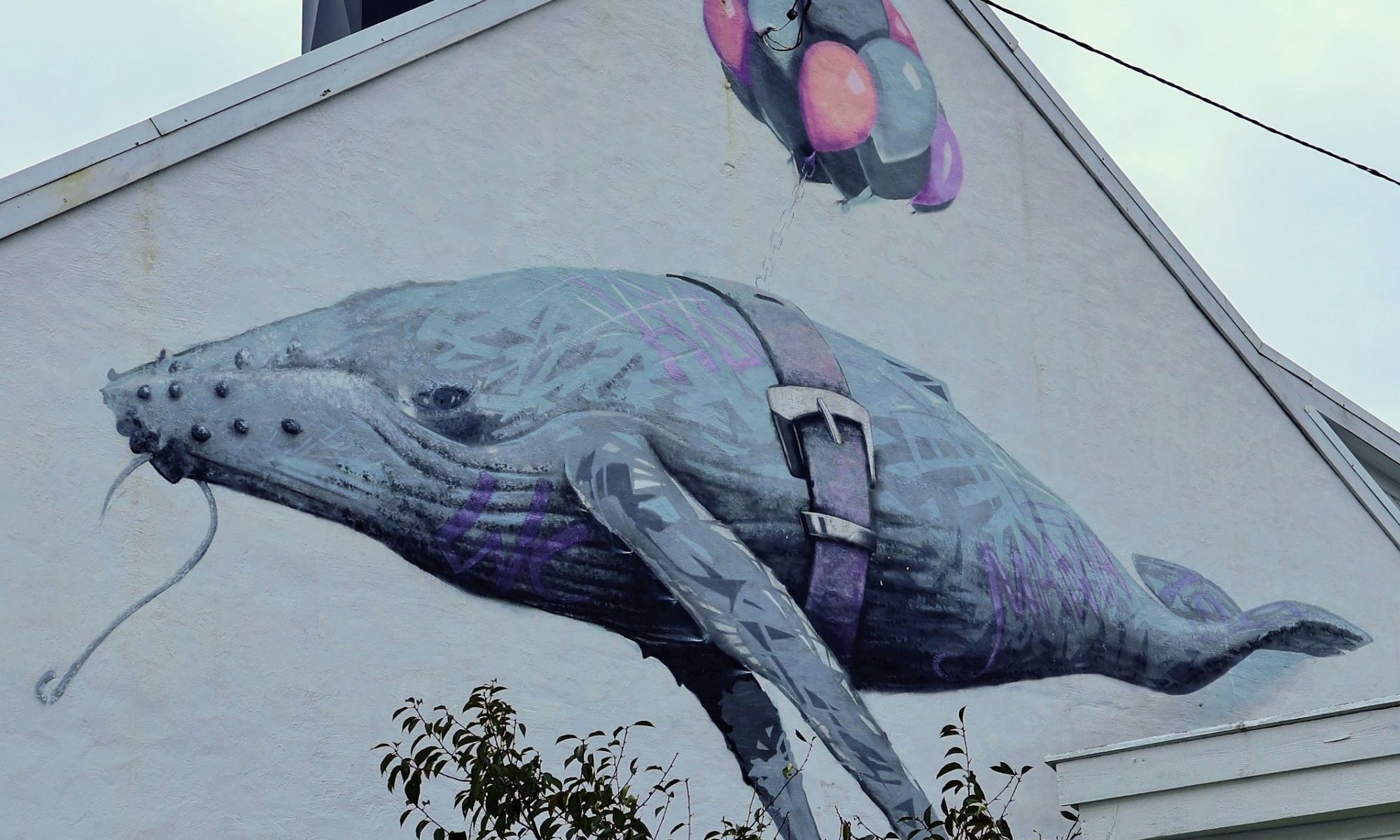This photograph captures a detailed mural painted on the side of a plain, light grey building with a steep roof that is cut off at the top of the frame. The mural features a mostly blue and grey whale with purple stripes and visible scarring on its back, which gives it a sense of past struggle or injury. The underside of the whale displays a striped pattern of grey and light blue, while its back is adorned with a black belt fastened by a silver buckle. From this belt, a small silver chain extends upwards, attaching to a colorful cluster of balloons in shades of orange, pink, purple, and light blue—colors that complement the whale's hues. The whale, which has a giant, curved hook piercing its lip, appears to be floating against a backdrop of a yellowish-blue sky. Beneath the mural, on the bottom of the frame, there is a small silhouette of leafy plant life, adding a touch of natural contrast to the scene. The overall pastel and subdued color palette of the mural makes it a striking and thought-provoking piece of art, possibly conveying deeper messages about freedom and entrapment.